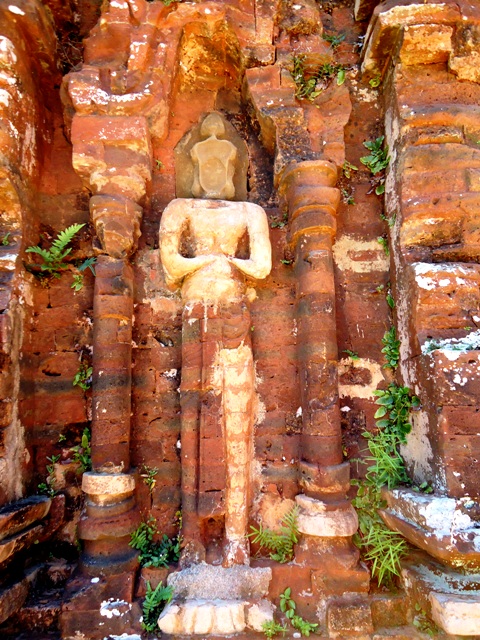The image depicts an ancient statue integrated into a crumbling temple structure made of red clay-colored bricks, suggesting it has been there for centuries. The statue, possibly representing a woman with arms crossed, is carved from a slightly different, white stone and stands amidst a messy, degraded temple environment. The temple, which might be Buddhist or Hindu, is encased in rocks and surrounded by lush, green plants. The setting is outdoor, marked by scattered debris, chalky fragments, and patches of moss and grass, adding to the impression of age and dilapidation. The statue itself features a distinct headpiece and is central to the temple’s ruins, hinting at its historic and cultural significance.